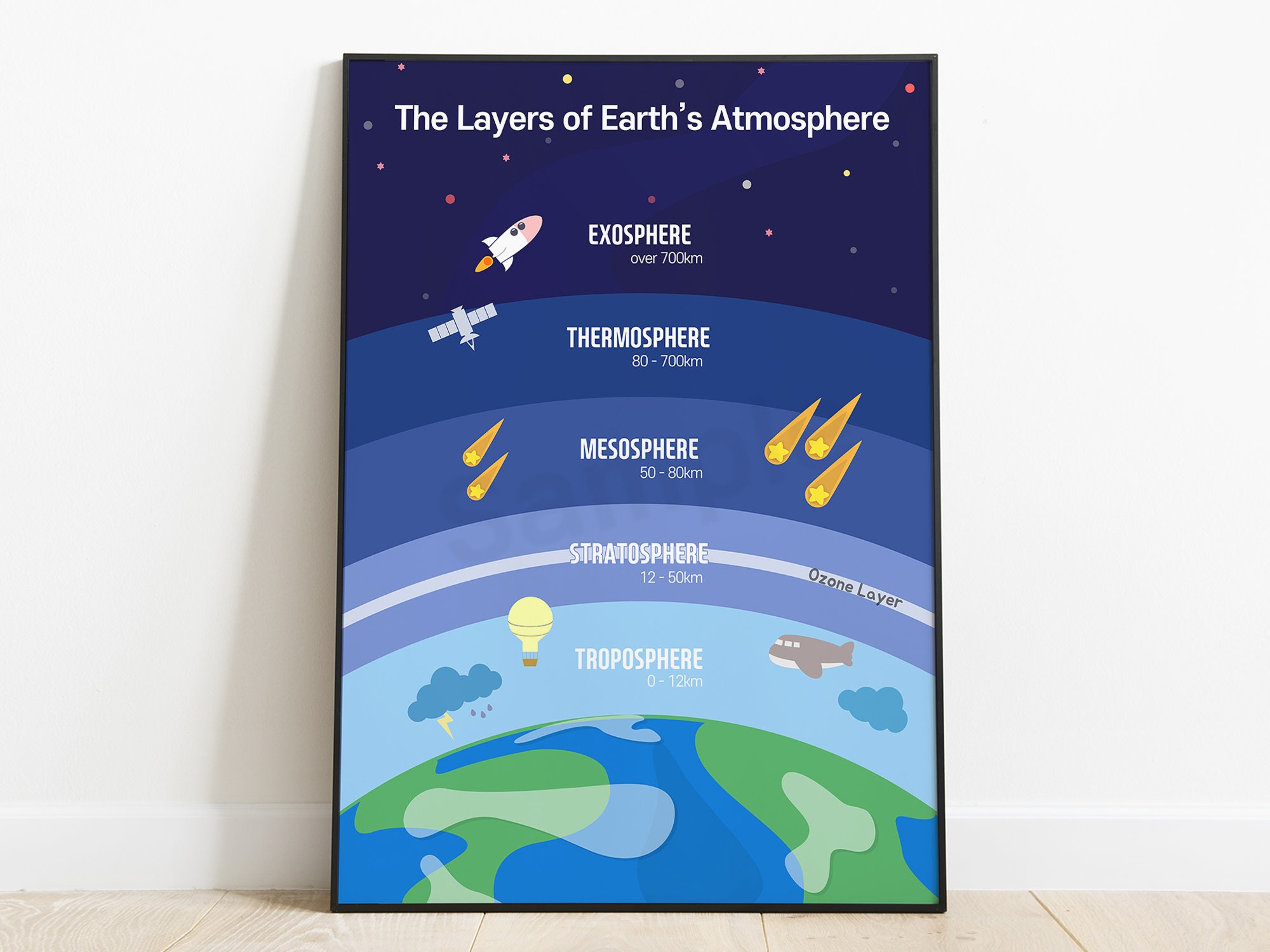This is an image of a detailed educational poster leaning against a white wall with a light wooden floor and white baseboard. The poster is framed in black and prominently features the layers of Earth's atmosphere, with each layer vividly illustrated and labeled in white text. At the top, against a backdrop of space with colorful stars, a rocket represents the exosphere, labeled "over 700 kilometers." Below that, the thermosphere is depicted in a lighter blue with a satellite and labeled "80 to 700 kilometers." The mesosphere is shown with meteors and spans "50 to 80 kilometers." The stratosphere includes the ozone layer and extends "12 to 50 kilometers." The troposphere, indicated by clouds, a hot air balloon, an airplane, lightning, and a thundercloud, covers "0 to 12 kilometers." At the very bottom, a semicircular representation of Earth showcases green landmasses, white clouds, and blue oceans. The poster's art style is naive and simplistic, making it an ideal educational tool for classrooms or other learning environments.